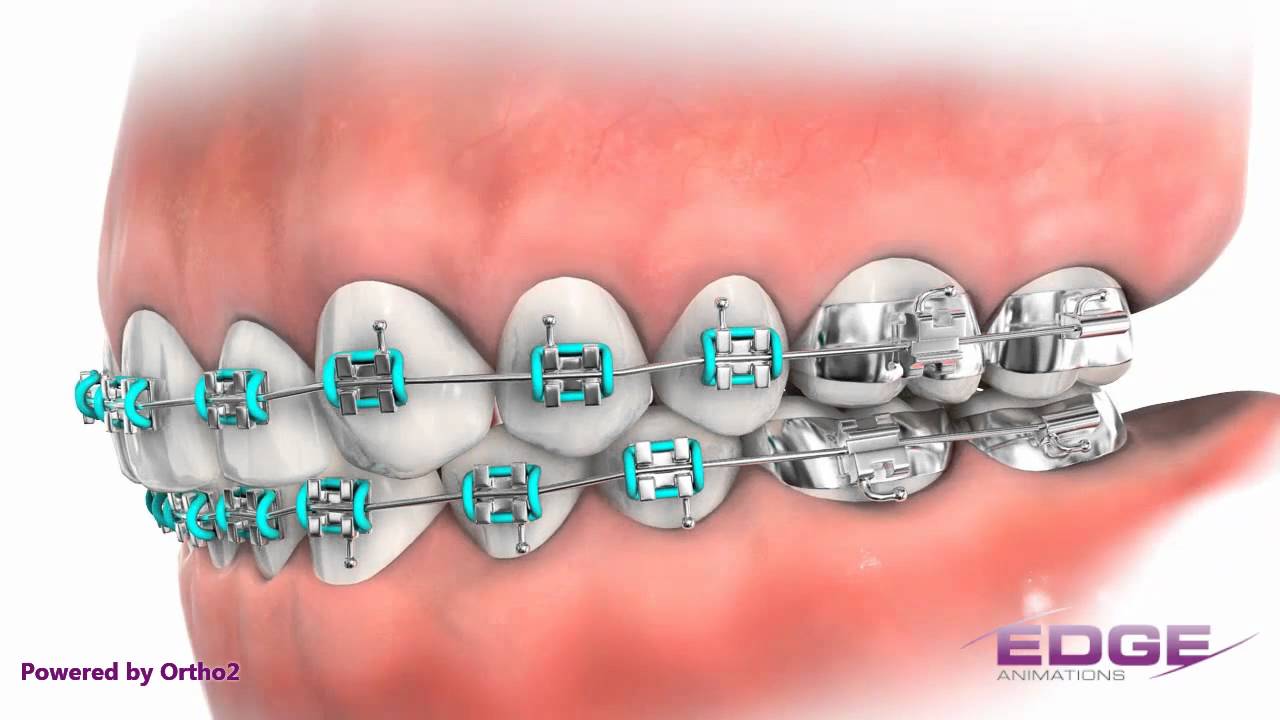This digitally rendered image showcases a detailed illustration of an open mouth featuring braces on both the upper and lower sets of teeth. Dominating the scene are the enlarged, pinkish-red gum lines, devoid of lips and other mouth parts, giving a close-up view of the orthodontic apparatus. The braces are distinctively characterized by turquoise-colored clamps attached to each tooth, connected by a metal wire running horizontally across the teeth. The molars at the back sport more substantial, stainless steel brackets that encase the teeth, likely designed to manage the tension of the bands more effectively. The image is bordered by text; "Powered by Ortho 2" appears in purple font in the bottom left corner, while "Edge Animations" is similarly placed in the bottom right. This detailed, computer-generated illustration provides an insightful look into the structure and function of braces within the mouth cavity.